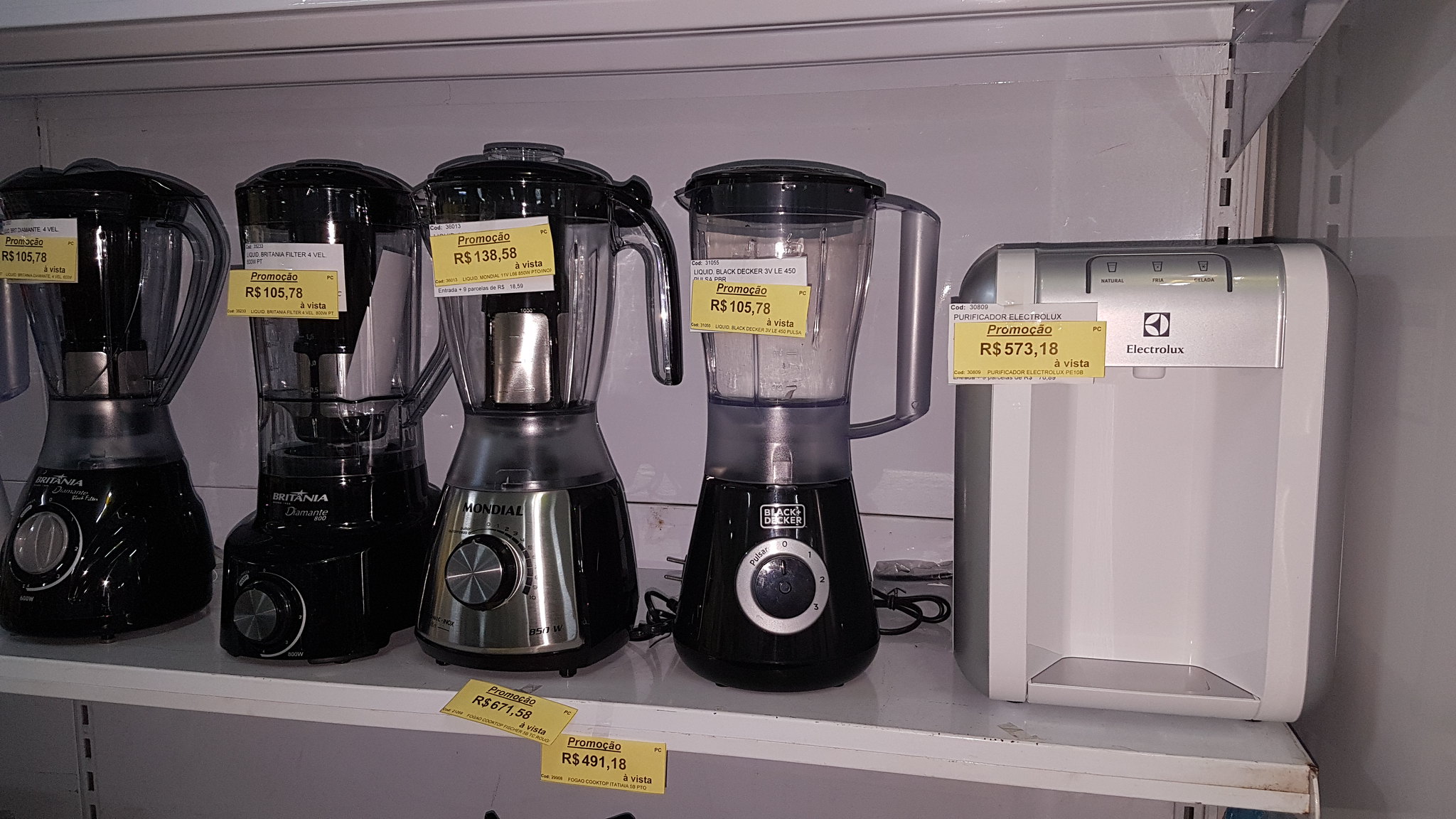This image appears to be taken in a store, perhaps a thrift shop or department store, showcasing a white metal shelf filled with kitchen appliances. The shelf prominently holds five products: four blenders and what seems to be a white, silver-edged coffee or tea maker, which some descriptions suggest might also be a purified water or ice machine. The coffee or tea maker is located on the far right, featuring a spot for placing a cup or glass, though no cup or glass is currently present.

From left to right, the shelf holds the following: the first blender, a black model with a dial handle; the second blender, similar in color, combining black and silver elements also with a dial; the third blender, completely black and also featuring a dial; and the fourth blender, which is black and has a silver plate at the bottom, labeled "Mondial." Each appliance has a yellow price tag, which is mounted on a white piece of paper, indicating promotions with the term "Promocito." The prices are marked in a currency signified by "R$", possibly Russian rubles. The tags on the shelf itself suggest further promotions.

While not explicitly clear if these products are new or used, one of the blenders appears to have a dirty knob, indicating potential prior use. The brand "Electrolux" is noted on one machine, adding a hint of authenticity and branding to the items displayed.